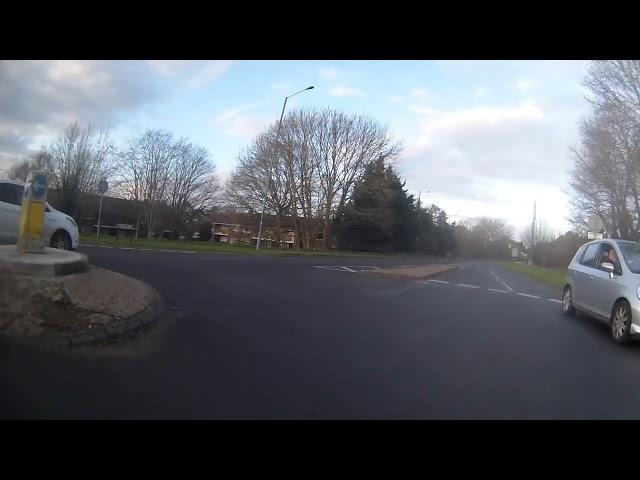A detailed aerial photograph captures a bustling intersection framed by black bars at the top and bottom. Dominating the bottom half of the image is a roundabout with a dark gray road surface. At its center is a cracked concrete circle with a smoother concrete protrusion capped by a distinctive yellow-and-white triangular bollard. Each white face of the bollard features a blue circle with a white left-pointing arrow, viewed from the photographer's perspective.

To the left side of the roundabout, a white car with black windows and tires navigates the roundabout, adhering to the left-hand traffic pattern. On the right side of the frame, partially out of view, a silver car drives in the bottom lane, its right passenger window open. The road extending from the roundabout features a dark red or brown median, dividing two lanes that stretch toward the horizon.

In the distance, left of the road, stand several wall-to-wall apartment buildings topped with black roofs. Leafless trees with branches fanning out in crown-like shapes line the avenue, their bare limbs reaching up starkly against the blue sky. Some similar trees are also present on the right side of the road. The scene is set beneath a sky mottled with gray and white clouds, adding to the crisp, urban aesthetic of the image.